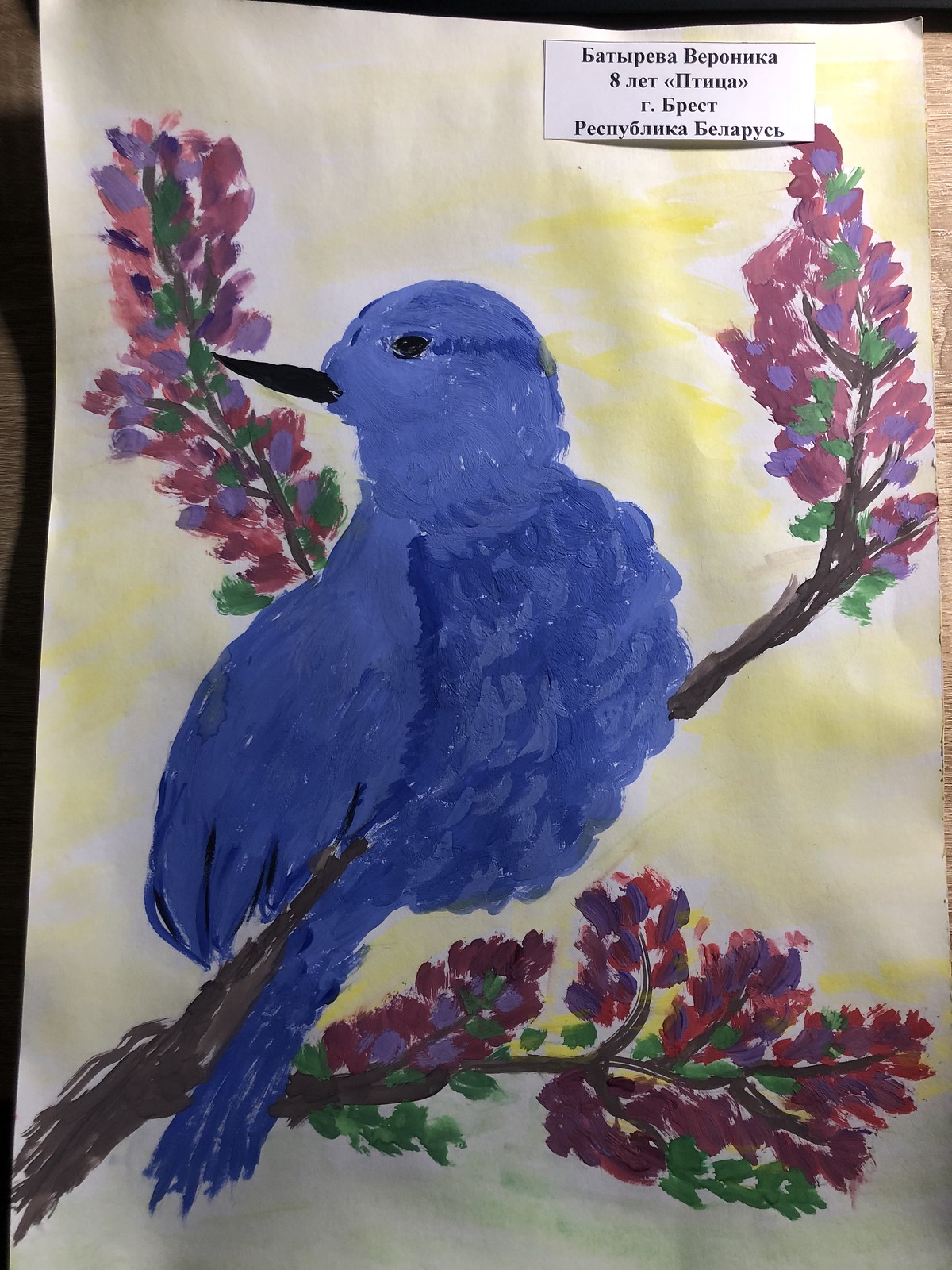An acrylic painting of a bluebird graces a piece of slightly wrinkled paper, which rests on a brown desk with just slivers visible to the left and right. In the upper right-hand corner of the paper, a rectangular label is affixed, displaying acrylic writing. The label includes a first and last name, the date, an initial with a dot and a word, and possibly two additional longer words at the bottom.

The bluebird, painted in variegated shades of blue, dominates the center of the paper, extending across approximately three-quarters of its width. The bird features a black beak and eye and is perched on a long brown branch, with its head turned to the left. Surrounding the bluebird are colorful blooms and small sprigs of green leaves. The branch itself has three main offshoots extending to the left, right, and center, with additional sprigs adorned with green leaves and vibrant red, purple, and pink blossoms. The background is a bright and cheerful yellow, making the bluebird and its floral perch stand out vividly.